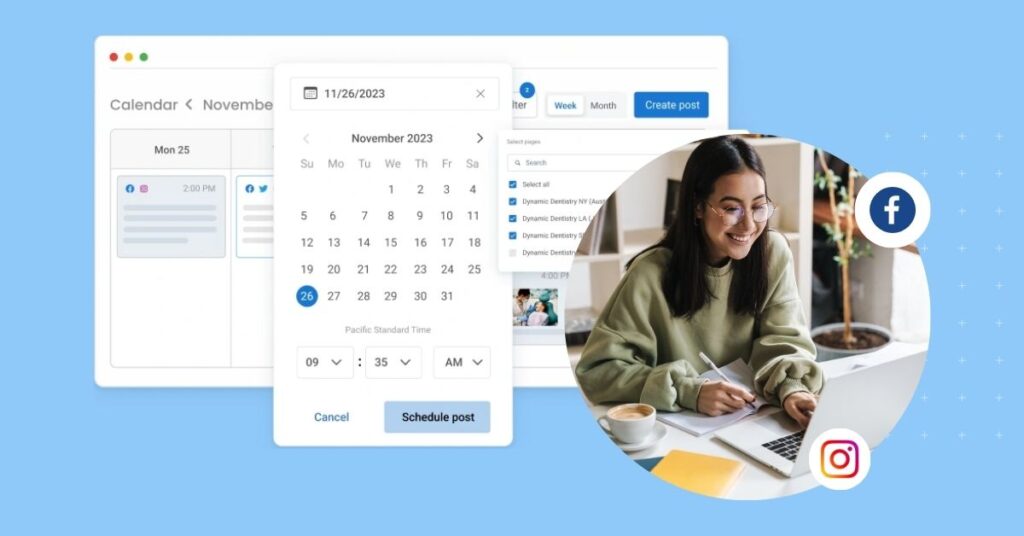The image features a light blue background with a large white square in the center. At the top left corner within this square are three small dots: red, yellow, and green. Directly below these dots is the word "Calendar."

Adjacent to the word "Calendar" is another term, "November," introducing a long white rectangle displaying a calendar icon and the date "11-26-2023." Beneath this rectangle, the text "November 2023" is written, followed by a full calendar layout for the month. The month starts on a Wednesday with the 1st and concludes with Thursday the 30th. Notably, Sunday the 26th is circled in blue, and beneath the calendar, the time "9:35 a.m." is specified. At the bottom, there are two button options: "Cancel" in a standard style and "Schedule Post" inside a blue box.

On the right side of the image, within a circular frame, is the photo of a young woman. She has black hair, wears glasses, is seated at a desk, and is working on a laptop. In front of her are a piece of paper, a pen, and to her left, a cup of coffee.

Additionally, in the upper right corner inside a small blue circle is the letter "F," representing the Facebook icon. Below this, within a white circle, is the pink and yellow camera icon symbolizing Instagram, indicating the sharing options to Facebook and Instagram, respectively.